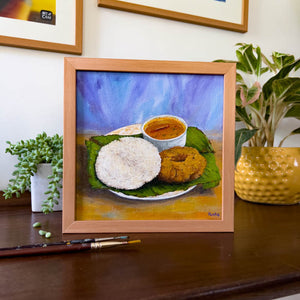The image depicts a deep brown wooden table with a polished surface, positioned alongside a white-colored wall. On the table, there is a small, square wooden frame containing an abstract artwork featuring a plate with a cup of liquid, a donut or bagel, and a round flatbread, set against a blue and purple background. Flanking the artwork are two potted plants: on the left, a cascading plant in a white, square pot, and on the right, a small plant with pink-tinged leaves in a light orangish, hammered round pot. Also on the table, in front of the artwork, are two paintbrushes. On the white wall behind the table, the bottom edges of two additional framed pictures can be seen.